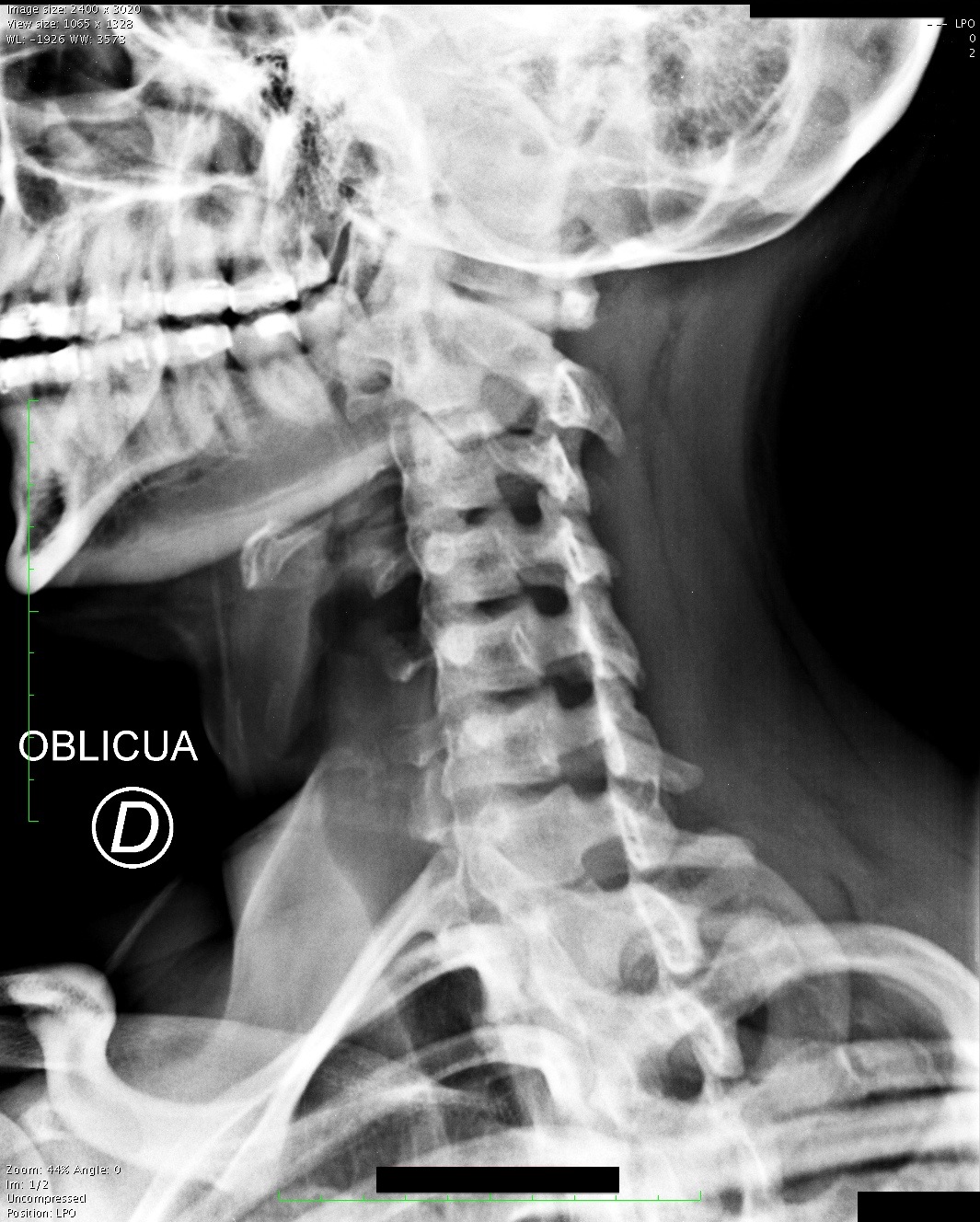The image is a detailed x-ray of a human head, neck, and upper torso, presented in a photographic style that mimics the appearance of a traditional x-ray. The central focus of the x-ray is the person's cervical vertebrae, which reveal the intricate structure of the neck's spine. The x-ray also captures the lower part of the skull, showcasing the teeth and the back of the skull, but notably, the eyes are not visible. The person appears to be facing left, providing a clear profile view of their head, shoulders, and upper ribcage.

The overall color scheme is a silver hue set against a black or gray background, which enhances the contrast and makes the skeletal details more discernible. Notable is the white text in the image which reads "O-B-L-I-C-U-A" with the letter "D" in a white font on a black circle with a white border below it, prominently located under the chin area. Additionally, on the left-hand side of the image, there’s text that reads "zoom 4% angle 0," followed by some unreadable black text and further information indicating "uncompressed position, LPG." The image also features two distinct black bars: one in the bottom right corner and another along the left side, which might be related to a hyoid bone fracture indicated by the dark bars.

This thorough depiction provides a comprehensive view of the anatomical regions captured in the x-ray, including the profile view of the neck and shoulders, and highlights the key textual annotations present in the image.